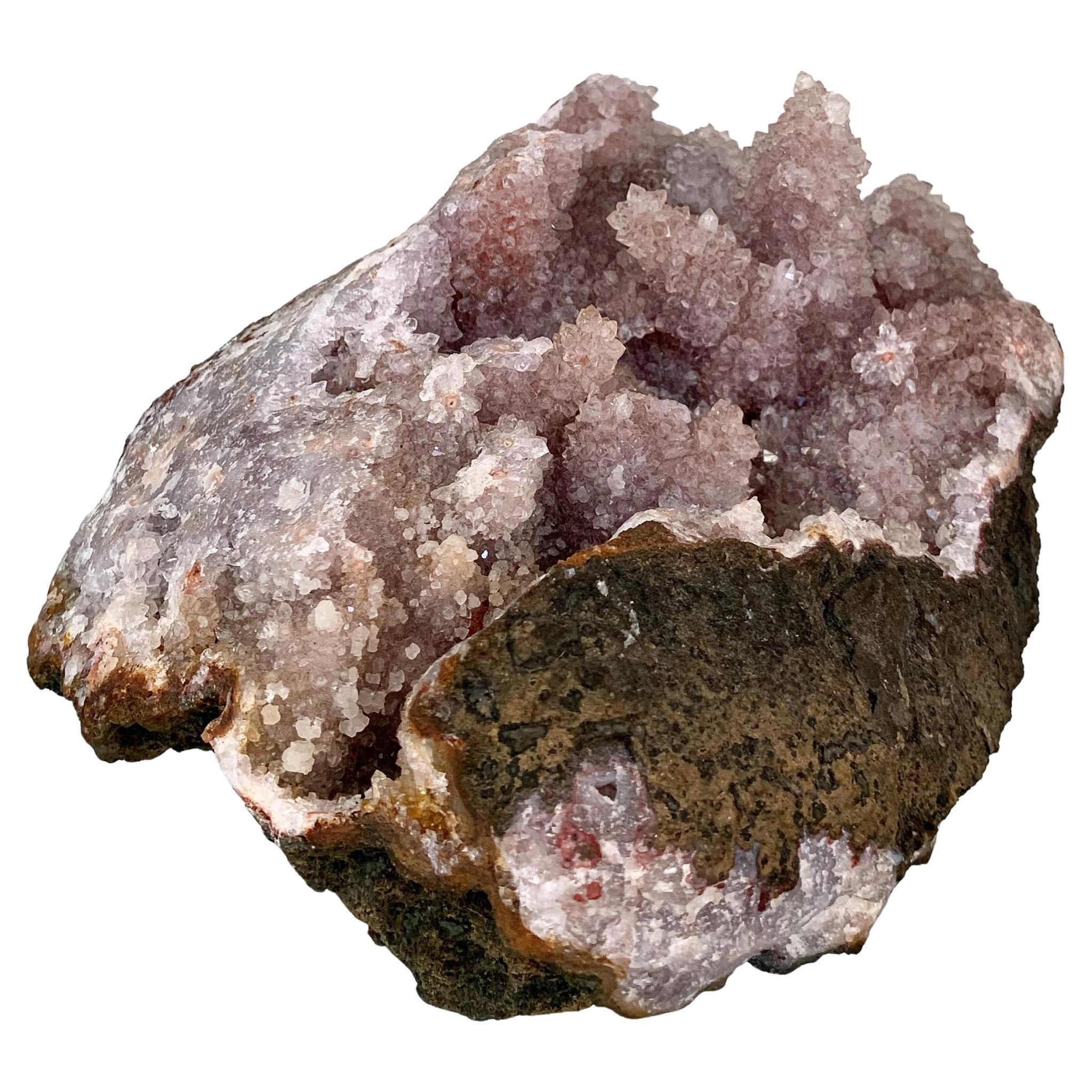The image depicts a halved amethyst geode, exhibiting a contrast between its rough, earthy exterior and its intricate, crystal-laden interior. The outer surface is an irregular, misshapen mix of brown and black, with occasional reddish speckles, conveying a rugged, natural appearance. In stark contrast, the interior reveals a stunning array of light purple, gray, white, pink, and red crystals, though the interior cavity is not overly hollow. The crystals do not exhibit a high shine; instead, they present a matte finish, allowing the subtle beauty of the geode's crevices and textures to be appreciated. The geode appears to be floating against a completely white, nondescript background, making it difficult to discern the geode's size or setting. The image is taken from a three-quarter view, providing a comprehensive glimpse into the depths and unique formations within this semi-precious stone.